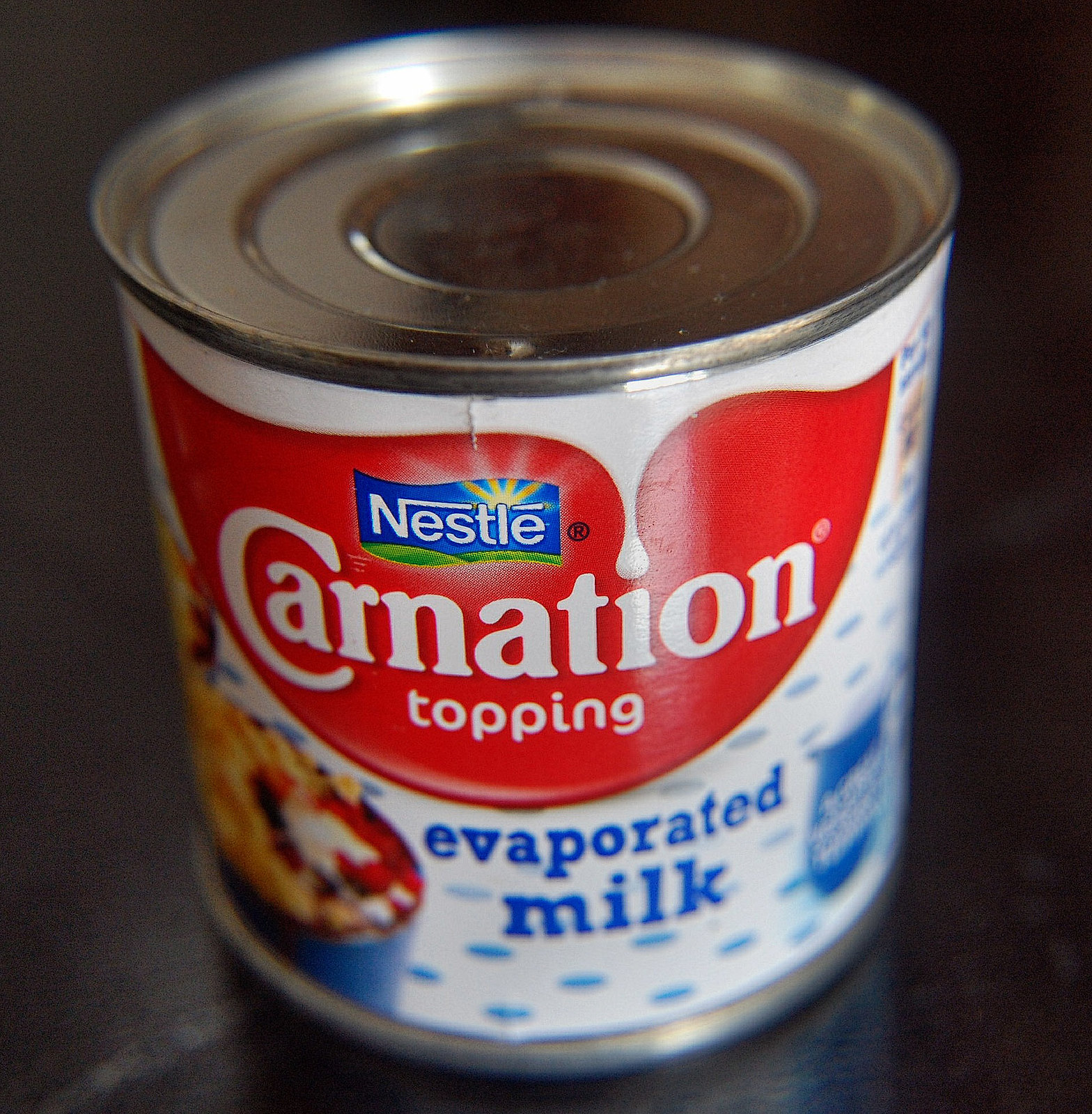The close-up image depicts a small, medium-sized can of Nestle Carnation Topping evaporated milk positioned on a slightly reflective black countertop. The can features a silver metallic finish with a prominent, shiny wrapper adorning its side. This wrapper is predominantly white, adorned with a large red dove-shaped graphic that contains the brand name "Carnation" in bold white text. Above this, a flag-shaped motif in blue and green displays the "Nestle" logo with a depiction of a blue sky, green hilly grass, and sunshine. Below the red section, in blue text, the label reads "evaporated milk." The white background of the label is interspersed with blue dots and specks, and there seems to be an image of a pie or dessert. The can's lid remains intact, and the image has a soft focus, giving it a slightly fuzzy border.